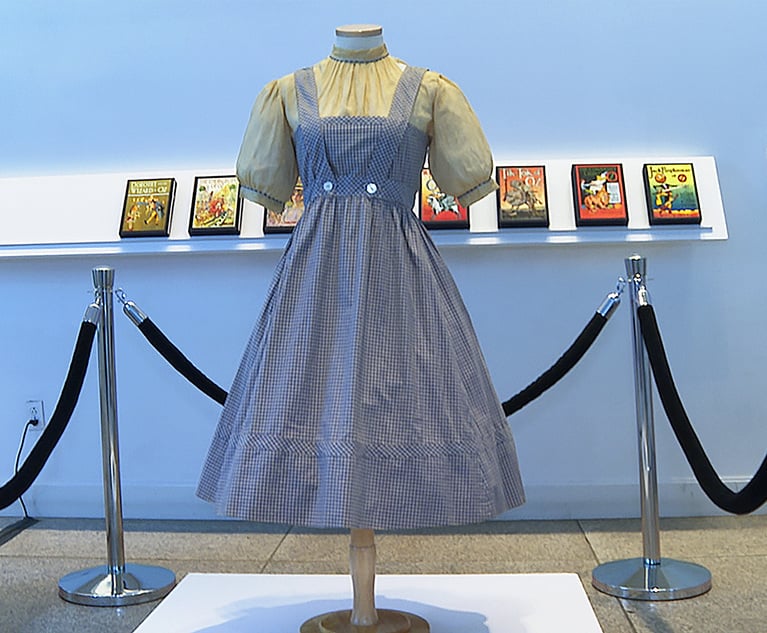The photograph depicts a museum exhibit showcasing a women's dress that strongly resembles the iconic blue gingham dress worn by Dorothy in "The Wizard of Oz." The dress is displayed on a headless and armless dress mannequin, set on a white pedestal with a wooden stand. The blue and white checkered dress features white buttons and is layered over a white short-sleeved blouse with blue stitching around the neck and sleeves. Black velvet ropes, held by stainless steel stanchions, section off the exhibit to prevent close contact. The backdrop includes a blue wall with a shelf at mid-level, holding a collection of colorful books or possibly poster arts related to the movie, although the specific images and texts are not clearly discernible. The floor beneath the exhibit is a glossy, gray stone tile, typical of an industrial or museum setting. The dress appears to have some wrinkles, adding to its authentic, lived-in look.